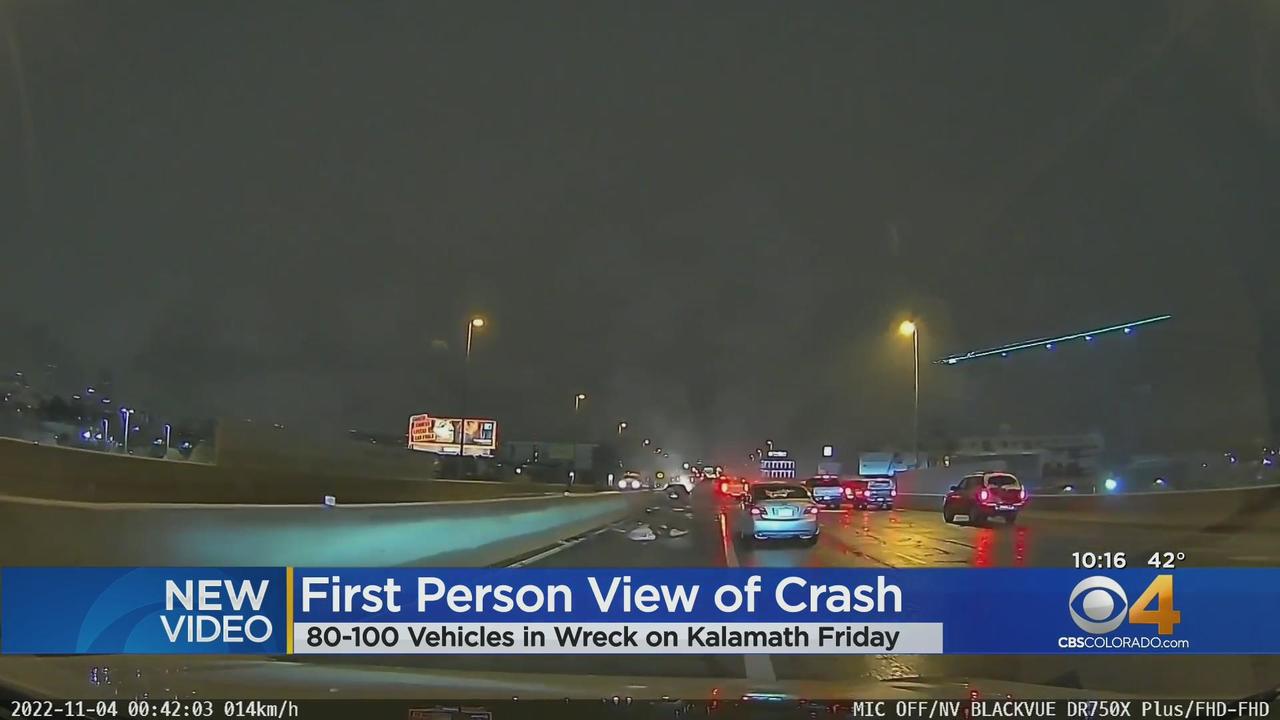The image is a detailed screenshot from a news broadcast on CBS Colorado, Channel 4, capturing a chaotic nighttime scene on a rain-soaked highway. The blue news banner at the bottom contains white text, stating "New video, first-person view of crash, 80 to 100 vehicles in wreck on Kalamath Friday." To the right, it also displays "1016, 42 degrees" with the CBS logo and the number 4. In the image, the sky is dark with streetlights positioned on the left and right sides illuminating the wet roadway. The highway appears cluttered; cars are stopped, some on the left shoulder, with evident crash debris. On the left side, there’s a wall dividing the lanes, and on the far left, a billboard is illuminated alongside some buildings and lights. The right side of the highway shows cars braking and trying to navigate the chaos. The top of the image is shrouded in mist from the rain, providing a somber, blurry backdrop. Along the very bottom, a black bar shows various data and technical details, further emphasizing the gravity and scale of the scene.